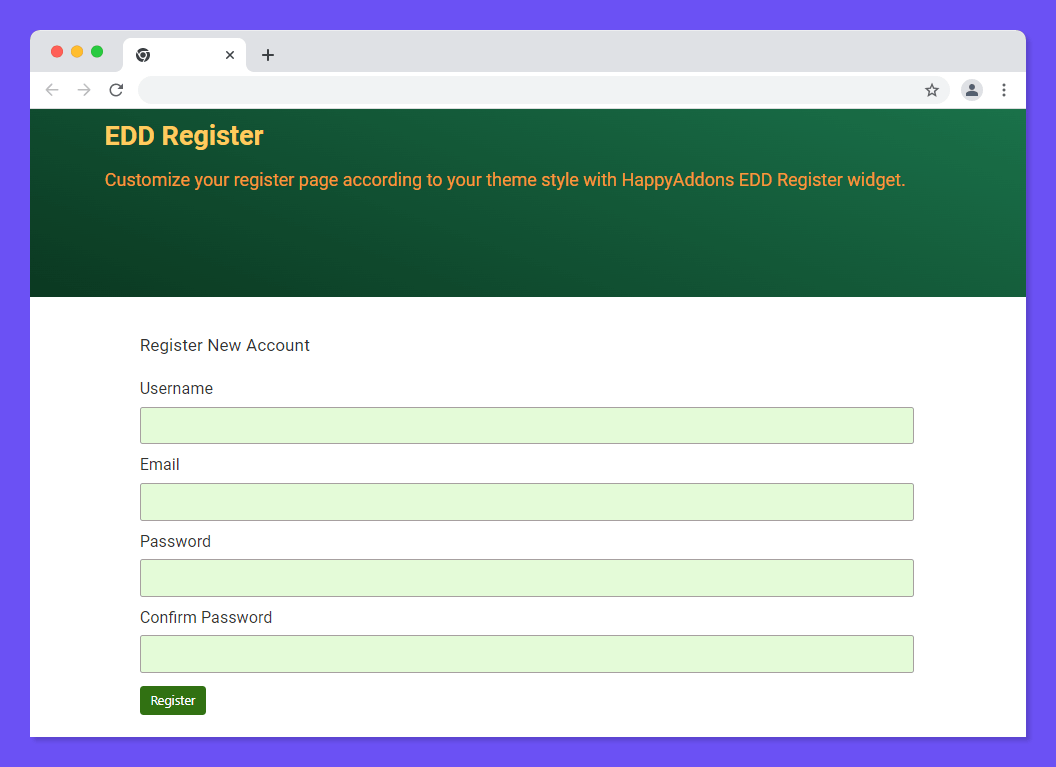The screenshot captures a desktop application window, bordered by a thick purple frame on all four sides. Within this frame, at the top-left corner, there are three colorful circular buttons—red, yellow, and a combined blue and green circle. Below these buttons, a large green horizontal section prominently displays the text "EDD Register" in yellow. Directly beneath that, in orange text, the message reads, "Customize your register page according to your theme style with Happy Addons EDD Register widget." Further down, against a white background, the form header states, "Register New Account." The form itself is positioned below this header.